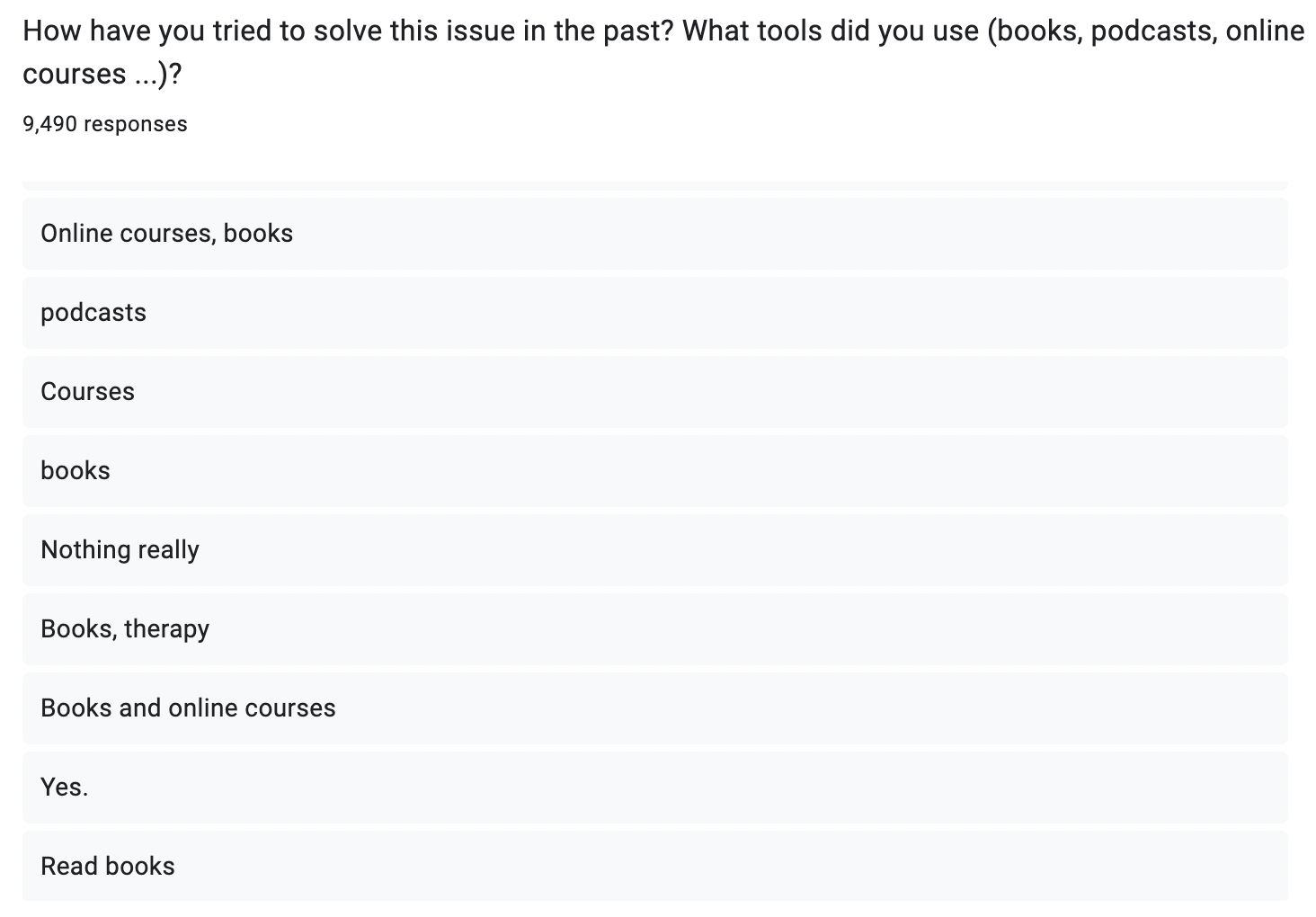The image is a screenshot of a webpage, likely from a survey site, given that it features a single question at the top. The page has a clean white background. The question, written in black text, asks: "How have you tried to solve this issue in the past? What tools did you use?" It includes examples such as books, podcasts, and online courses, and concludes with a question mark. Below the question, there is information indicating that there have been 9,490 responses. The response options available for selection are a mix of multiple-choice entries, including: "Online courses, books," "Podcasts," "Courses," "Books," "Nothing really," "Books, therapy," "Books and online courses," "Yes," and "Read books." Respondents can select one or multiple options that apply to their particular situation.